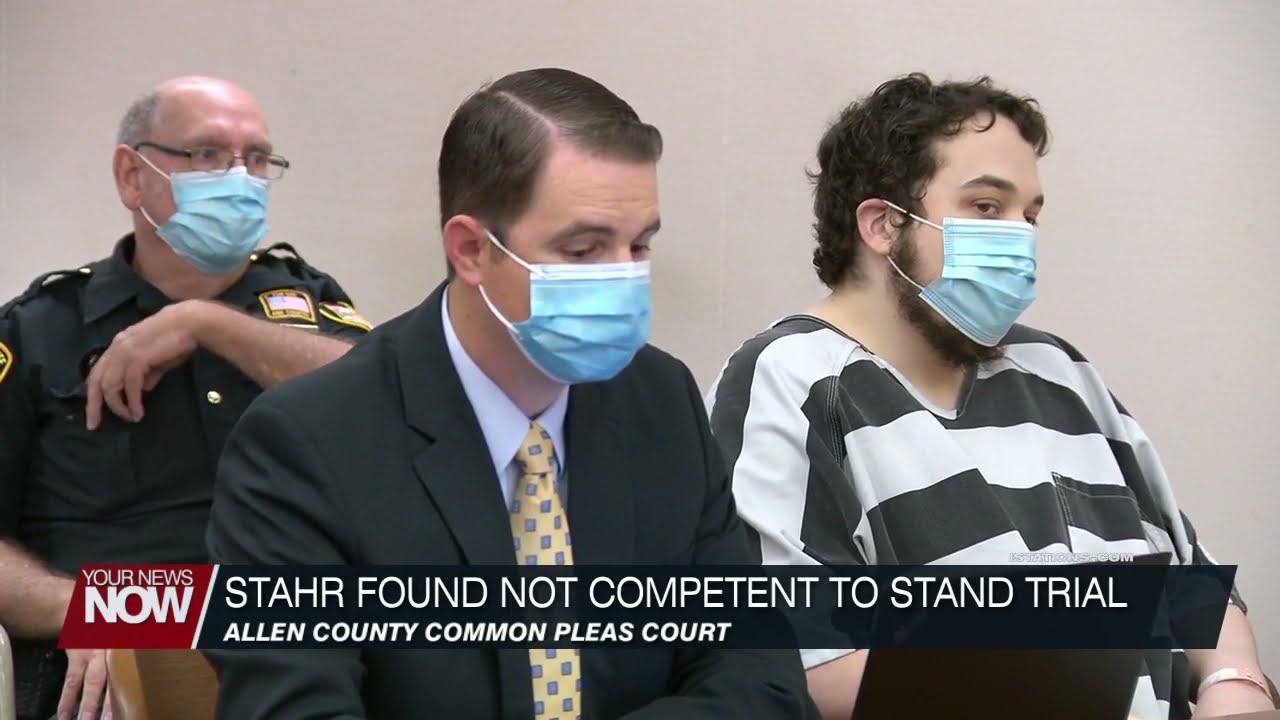This newsreel still image depicts a courtroom scene with three men who are all wearing blue medical masks. At the back, on the left, is a police officer in a black police uniform adorned with white and gold patches; he also wears glasses. In the front, on the left, is a lawyer dressed in a black suit featuring a light blue dress shirt and a yellow tie with a blue square pattern. Next to him, on the right, sits his client, a man in a black and white striped prison jumpsuit with short curly hair. The backdrop is a cream-colored wall typical of indoor courthouse settings. In front of the lawyer is a computer. The on-screen text includes the caption "Your News Now," with "Now" in larger, bolded letters. Below is a black box containing the text: "Star found not competent to stand trial," followed by an italicized line that reads "Allen County Common Pleas Court."